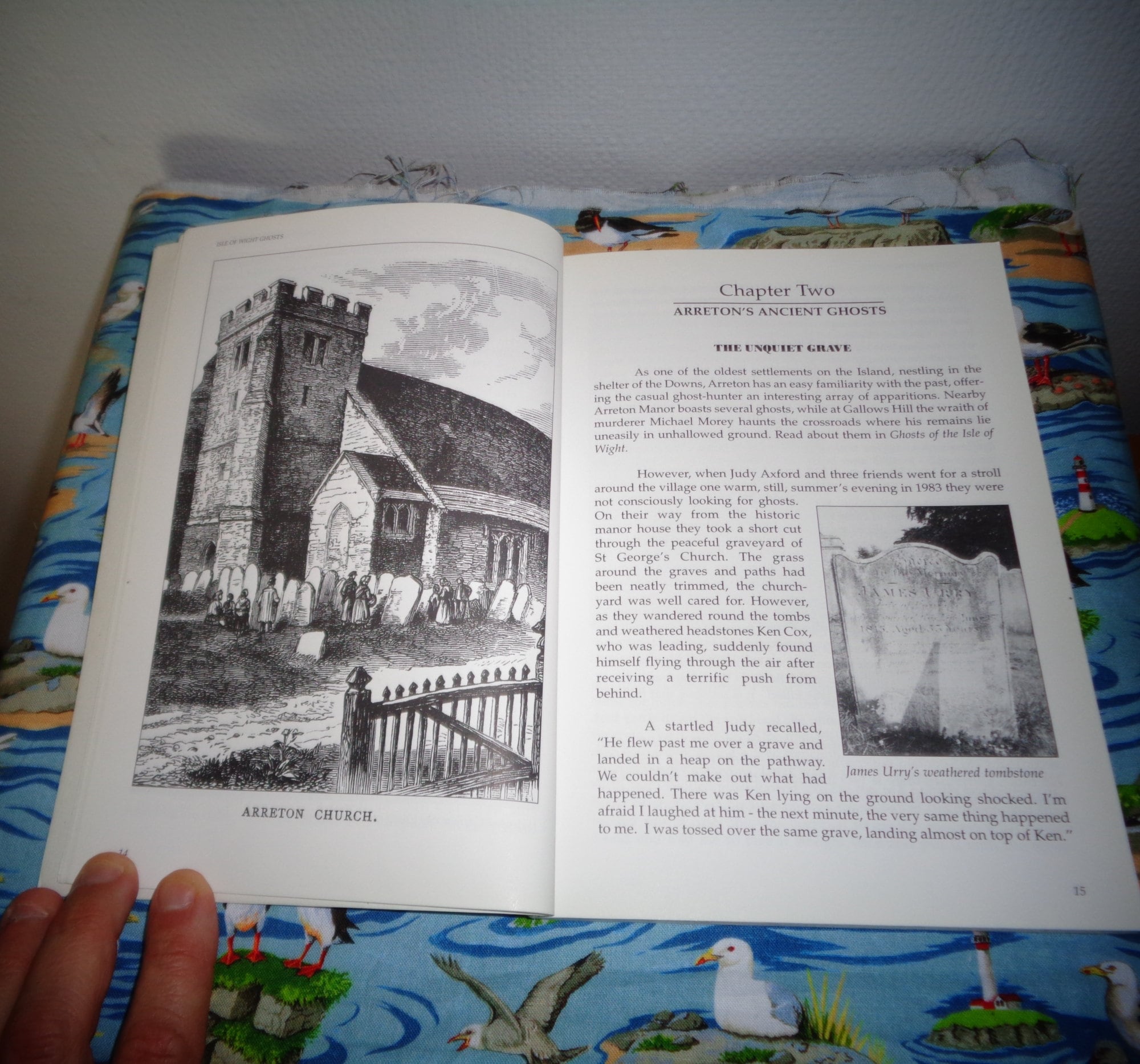The image features an open book set on a blue tablecloth that mimics water, adorned with a flying dove, green island, seagulls, and a lighthouse. The left page of the book displays a black and white illustration of an old-style church, identified as Arrington Church, which includes castle-like features, a graveyard with several gravestones, a road, and a fence. The right page, marked by a hand holding the book open with three fingers, announces Chapter 2 titled "Ayrton's Ancient Ghosts: The Unquiet Grave," followed by a passage of text. There is a smaller black and white image of a gravestone at the bottom of this page. The setting background is described as colorful, contrasting with a predominantly blue theme and fair complexioned fingers visible in the left corner.